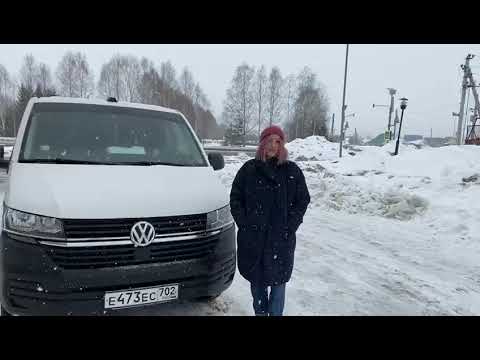In the middle of a winter scene, a woman is standing directly in front of a white Volkswagen van, identifiable by its prominent silver logo. The scene indicates a recent snowstorm or active snowfall, as evidenced by dense white snow covering the ground and large piles of snow in the background. The woman's attire reflects the cold conditions; she is dressed in a navy blue winter coat, blue jeans, and a red beanie, with her hands tucked into her coat pockets. Her hair, which appears to be either pinkish or blonde, drapes over her shoulders. The van's bumper is black, contrasting with its white body. She stands centered in the image, set against an industrial or urban backdrop featuring leafless trees, light posts, and possibly a factory, suggesting a location consistent with Germany or Europe. The parking lot where she stands appears recently plowed, with visible streets and posts embedded in the snow. The photograph captures a serene moment amidst a snowy landscape, with the woman looking calmly at the camera amidst drifting snowflakes.